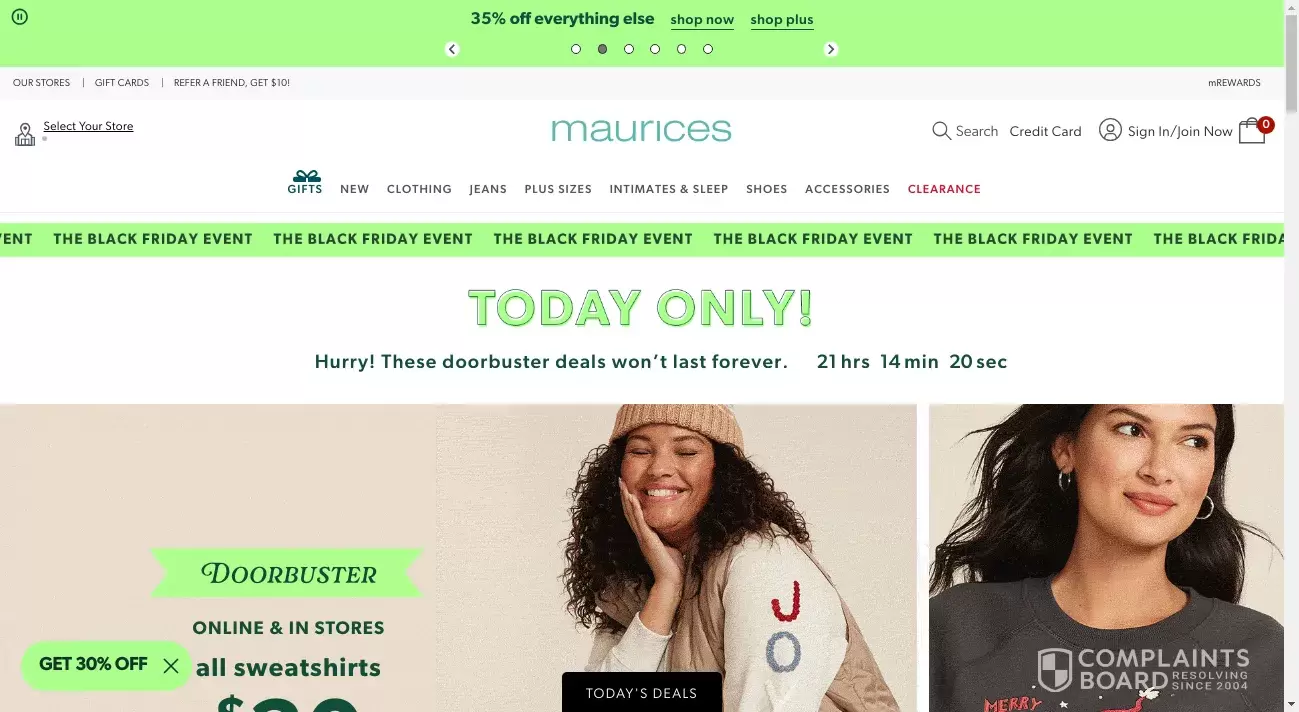The image depicts a computer screen with a pop-up advertisement from Marisa's overlaying the desktop background, which is partially obscured but features a sky view with visible trees in the bottom left and right corners. The desktop background appears to have some black text and a blue border at the top. The pop-up ad prominently displays a picture of two females standing in front of a white house, both wearing white t-shirts. The female on the left is dressed in blue jeans, while the female on the right is wearing green pants. The left side of the pop-up has a light blue background with the Marisa's logo at the top, followed by the text "Unlock 30% Off Your Order." Below this, there is a white input bar for an email address and a blue button that says "Sign Up and Save." In the bottom right corner of the advertisement, there is text that reads "Complaints Board: Resolving Since 2004," accompanied by a shield made up of white and black squares.